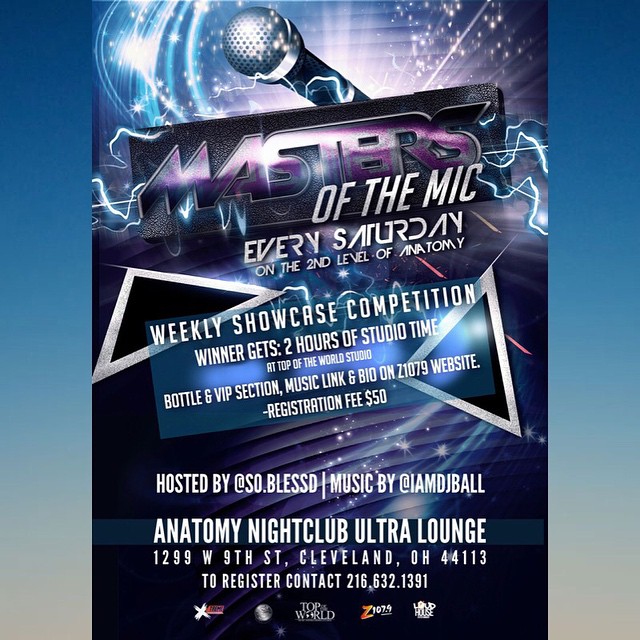This is a promotional card for Anatomy Nightclub Ultra Lounge in Cleveland, Ohio, designed to draw customers to their weekly event. The card features a dark blue border that fades to light blue, and then to beige on the left and right edges. At the top center of the card, a microphone is surrounded by stars and light reflections. Below this, in bold stylized block letters, are the words "Masters of the Mic," followed by "EVERY SATURDAY ON THE SECOND LEVEL OF ANATOMY" in white capital letters against a black background. 

The middle section of the card has a complex silver and dark background with reflected light and triangles, housing the text "WEEKLY SHOWCASE COMPETITION." The potential rewards for participants are listed: "Winner Gets: TWO HOURS OF STUDIO TIME at Top of the World Studio, BOTTLE & VIP SECTION, MUSIC LINK AND BIO ON Z107.9 WEBSITE." It also states the "REGISTRATION FEE: $50" in a smaller font below this.

The bottom section features the details of the hosts and location. In capital letters, it states "Hosted by @So.BlessD / Music by @IAmDJBall." Below this, "ANATOMY NIGHTCLUB ULTRA LOUNGE" is prominently displayed, followed by the address "1299 West 9th Street, Cleveland, OH 44113" in smaller text. Finally, it includes the registration contact details "To register, contact 216-632-1391" and several logos associated with the radio station Z107.9 and other partners.